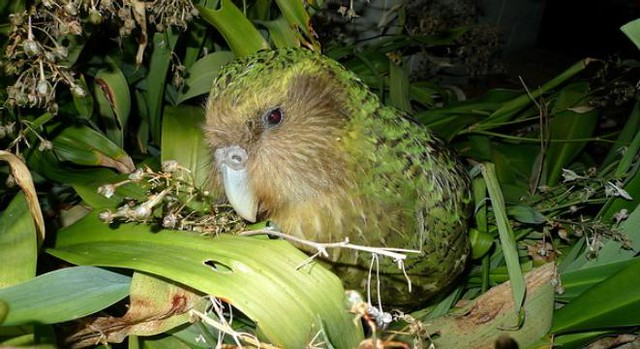The color photograph captures a close-up of a small bird nestled in a grassy setting, surrounded by various shades of green foliage that provide excellent camouflage. The bird, predominantly green with some black and yellow accents, features a head slightly turned towards the camera, revealing only its left eye, which has a subtle glow. The bird's face is adorned with light brown feathers, transitioning to a green body with hints of darker shades. Its beak is ivory-colored. The scene is brightly illuminated, likely by a camera flash, as the background fades into darkness, suggesting a nighttime environment. Long, leafy plants and sticks contribute to the natural, jungle-like appearance of the setting. The bird's position and environment hint at an unusual nesting behavior specific to its species.